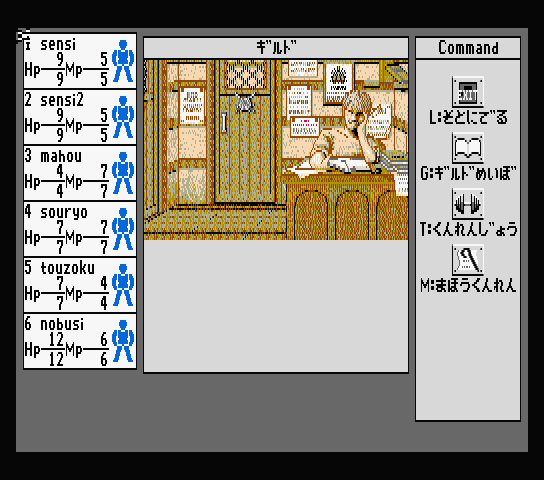The image is a color screenshot from an old computer game, characterized by its pixelated graphics. At the center of the image, a person is depicted sitting at a desk, facing forward with their right hand propping up their head. To the left of this central figure, there is a vertical list featuring six entries, each starting with the term "Sensei" followed by a unique name: Sensei 1, Sensei 2, Mahou, Soryu, Tezuku, and Nobuse. Each entry is accompanied by a small, blue illustration of a person with hands on their hips. 

Adjacent to each name, there are numerical values indicating health points (HP) and mana points (MP), which vary as follows: Sensei 1 - HP 9/9, MP 5/5; Sensei 2 - HP 9/9, MP 5/5; Mahou - HP 4/4, MP 7/7; Soryu - HP 7/7, MP 7/7; Tezuku - HP 7/7, MP 7/7; Nobuse - HP 4/4, MP 12/12. 

On the right side of the screen, near the top, the word “Command” is displayed, below which are various icons or symbols resembling letters, code, or hieroglyphics.

This intricate and nostalgic game interface is a testament to the early era of computer gaming with its basic yet engaging design elements.